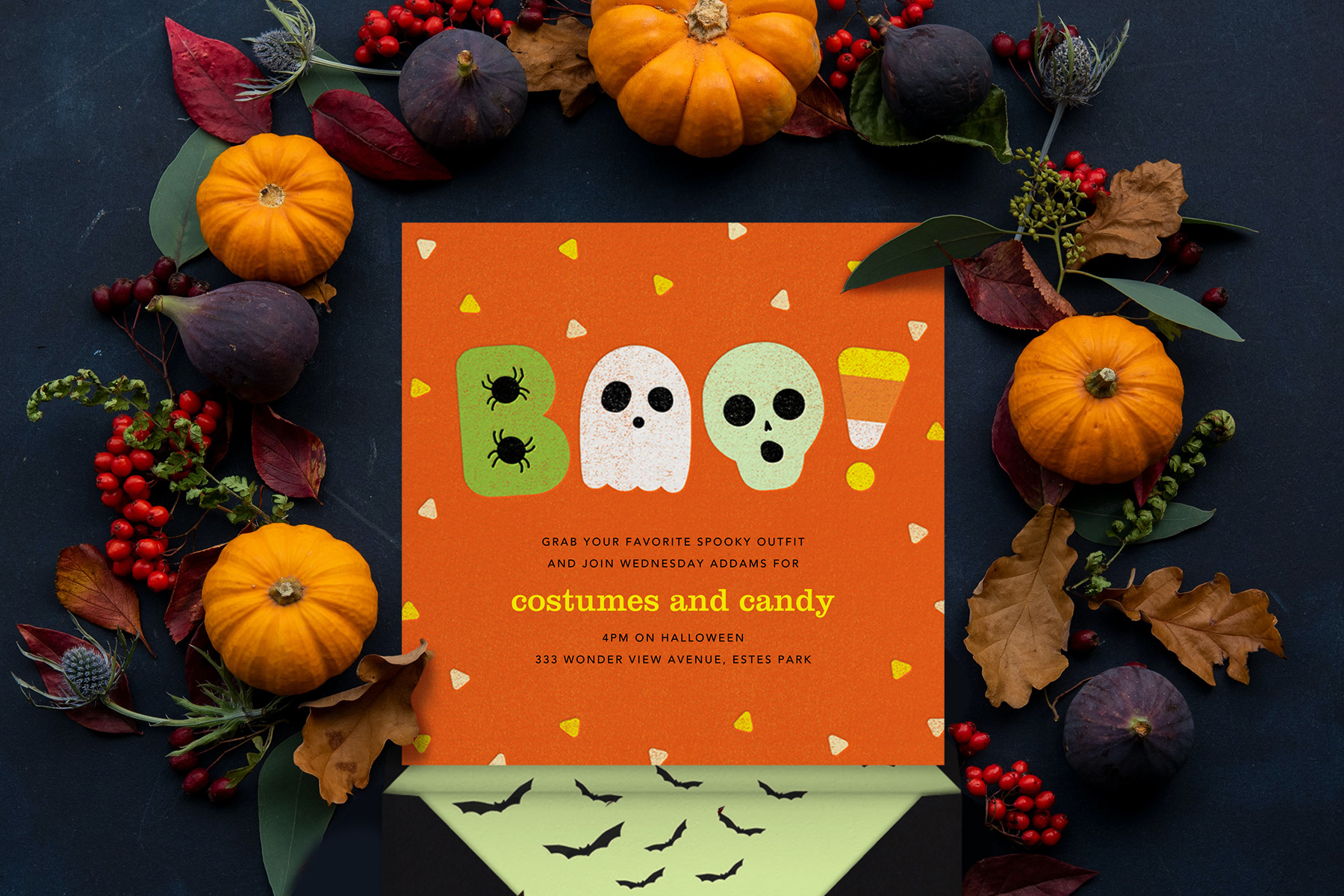A carefully staged, full-color photograph showcases a Halloween-themed table setting on a blue tablecloth. At the center of the scene is an orange card adorned with colorful, whimsical Halloween details. The word "Boo" is prominently displayed on the card, with a green "B" featuring spider details, a white ghost for the first "O," and a grayish skeleton for the second "O." The exclamation point is creatively represented by a candy corn. The card's background is dotted with small, multicolored triangles adding to its festive feel.

The card invites viewers to "grab your favorite spooky outfit and join Wednesday Addams for costumes and candy," with the invitation text in black and yellow. It specifies the event will take place at 4 p.m. on Halloween at 333 Wonderview Avenue, Estes Park. Surrounding the card, a variety of small baby pumpkins, dried leaves, berries, and other fall decor are artfully spread across the table, enhancing the seasonal ambiance. The entire arrangement is set against a square frame, bathed in the even glow of artificial indoor lighting.